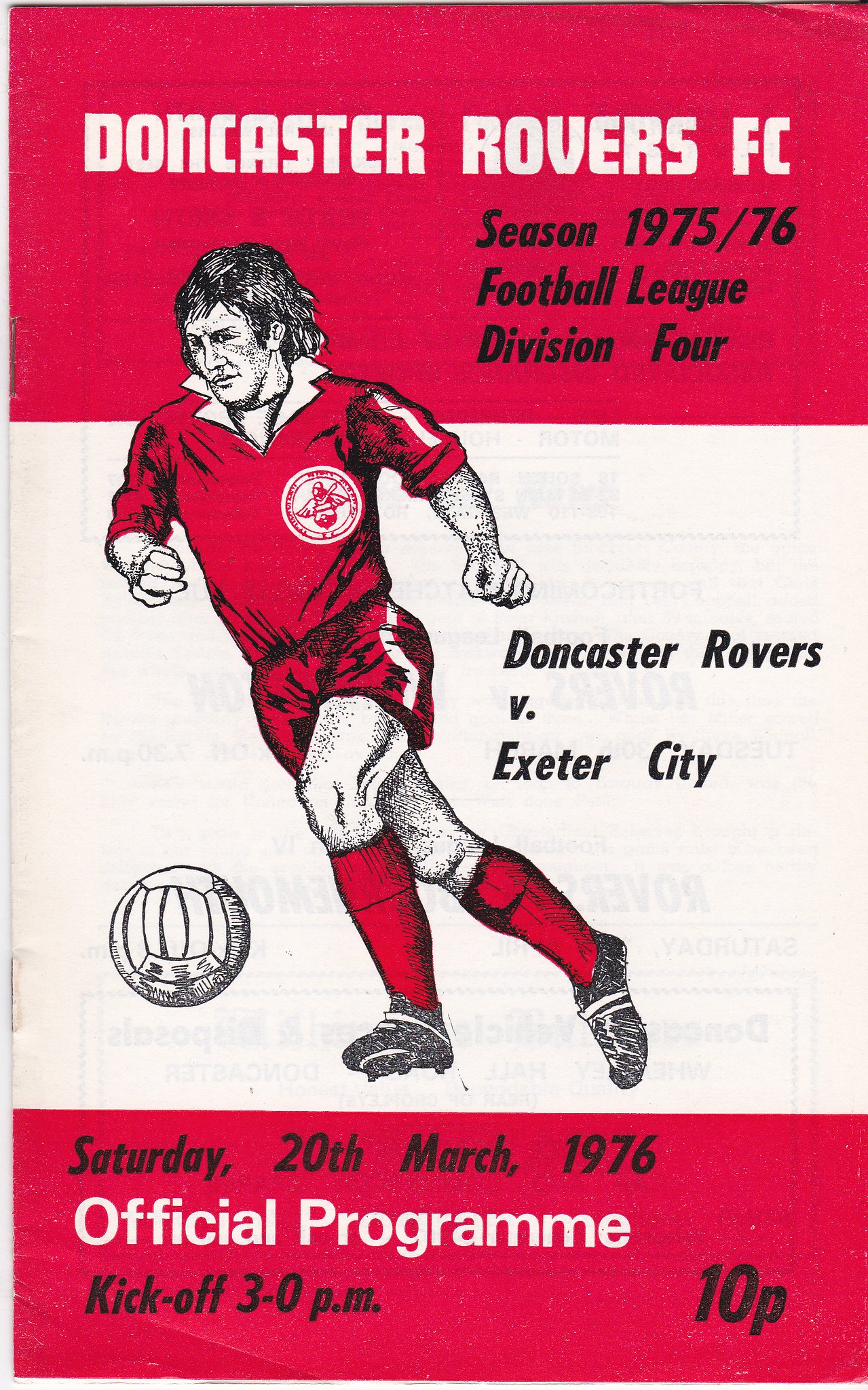This image is a cover for a program of Doncaster Rovers FC for the Season 1975-1976, in Football League, Division 4. It prominently features an illustration of a football player in a dynamic pose, chasing after a ball. The player is dressed in an all-red kit with white stripes along the sides of the sleeves and shorts, complemented by red socks and soccer cleats. His medium-length hair touches his shoulders, giving a sense of movement and energy.

The background is divided into three horizontal sections: the top third is a bold red color block, the middle section is white, and the bottom quarter is another red color block. The top red section includes white text that reads "Doncaster Rovers FC," with "Season 1975-76, Football League, Division 4" written in black underneath. The white middle section features the matchup information, stating "Doncaster Rovers vs. Exeter City." In the bottom red section, in black text, it says "Saturday, 20th March 1976," followed by "Official Program" in white text. Below that, in black text, it indicates the kickoff time "3-0 PM," and at the bottom right corner, it shows the price "10p" in white text. The overall color scheme is red, white, and black, giving it a classic and eye-catching appearance.